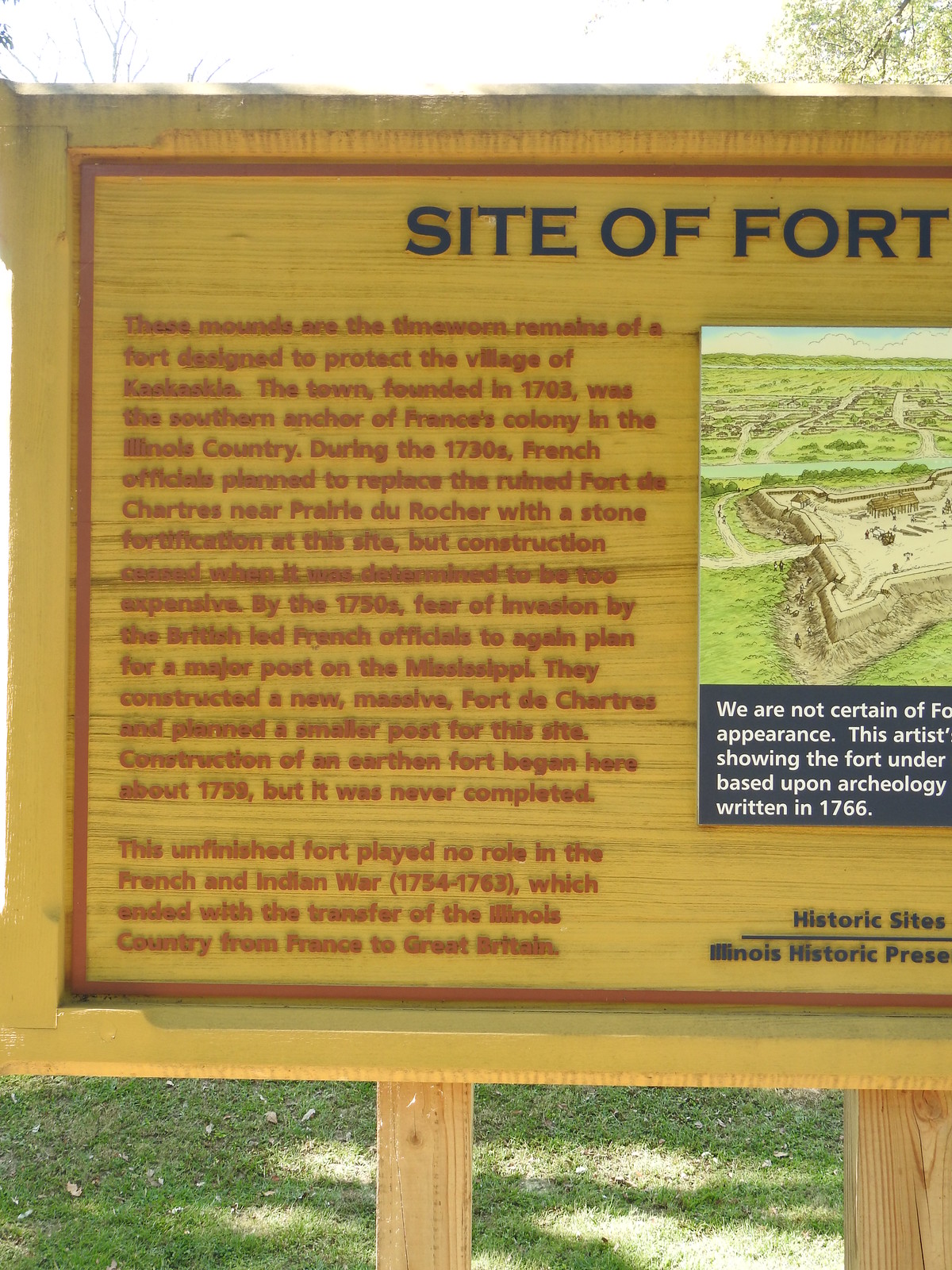The image showcases a large, relatively new wooden sign positioned outdoors, with fresh wood supported by two sturdy wooden posts surrounded by sun-dappled grass on both sides. The wooden sign serves as an informational plaque typical of historical sites or state parks. The background of the sign is a yellowish hue, and it features detailed textual and graphical information.

At the top, in black lettering, the sign reads "Site of Fort." Below, the text in orange explains the historical significance: "These mounds are the time-worn remains of a fort designed to protect the village of Kaskaskia. The town, founded in 1703, served as the southern anchor of France's colony in the Illinois country. During the 1730s, French officials planned to replace the ruined Fort de Chartres near Prairie du Rocher with a stone fortification here, but construction ceased due to expense. By the 1750s, fears of a British invasion prompted new plans for a major post on the Mississippi. Although construction of an earthen fort began around 1759, it was never completed and played no role in the French and Indian War (1754-1763), which ended with the transfer of the Illinois country from France to Great Britain."

On the right side of the sign, there is a color illustration depicting a map and image of the historic site, which includes green areas representing the landscape, a waterway, and the fort layout. At the bottom of the sign, the text reads "Historic Sites, Illinois Historic Preservation," signifying its placement at a preserved historic location.